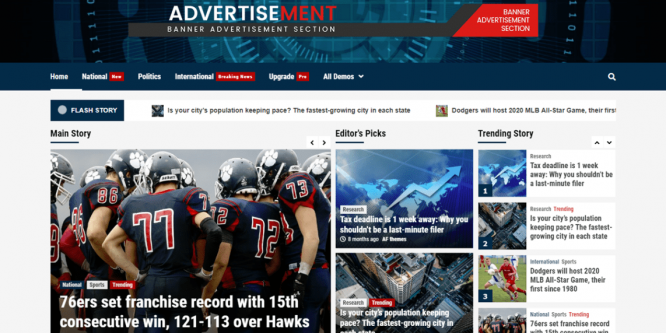This image is a screenshot in landscape mode of a website. The upper portion from left to right features a banner advertisement section, labeled "Advertisement Banner Advertisement Section" on the left and "Banner Advertisement Section" on the right, indicating where banner ads could be placed by the website owner.

Below the advertisement section, there is a dark blue navigation bar that includes tabs labeled "Home," "National," "Politics," "International," and "Upgrade." The "Home" tab is selected. The "National" tab has a red button next to it labeled "New," the "International" tab has a red button labeled "Breaking News," and the "Upgrade" tab has a red button labeled "Pro." It’s unclear whether these red buttons are clickable or simply indicators.

In the next section, the upper left-hand corner displays "Flash Story" and includes headlines such as "Is Your City's Population Keeping Pace?" and "The Fastest Growing City in Each State." Additionally, the headline "Dodgers Will Host 2020 MLB All-Star Game" is visible.

Below that, different sections are organized: the main story features the "76ers," accompanied by images. The "Editor's Picks" section highlights the "Tax Deadline" and other notable stories. The "Trending Stories" section displays rows of trending articles, providing an array of news topics.